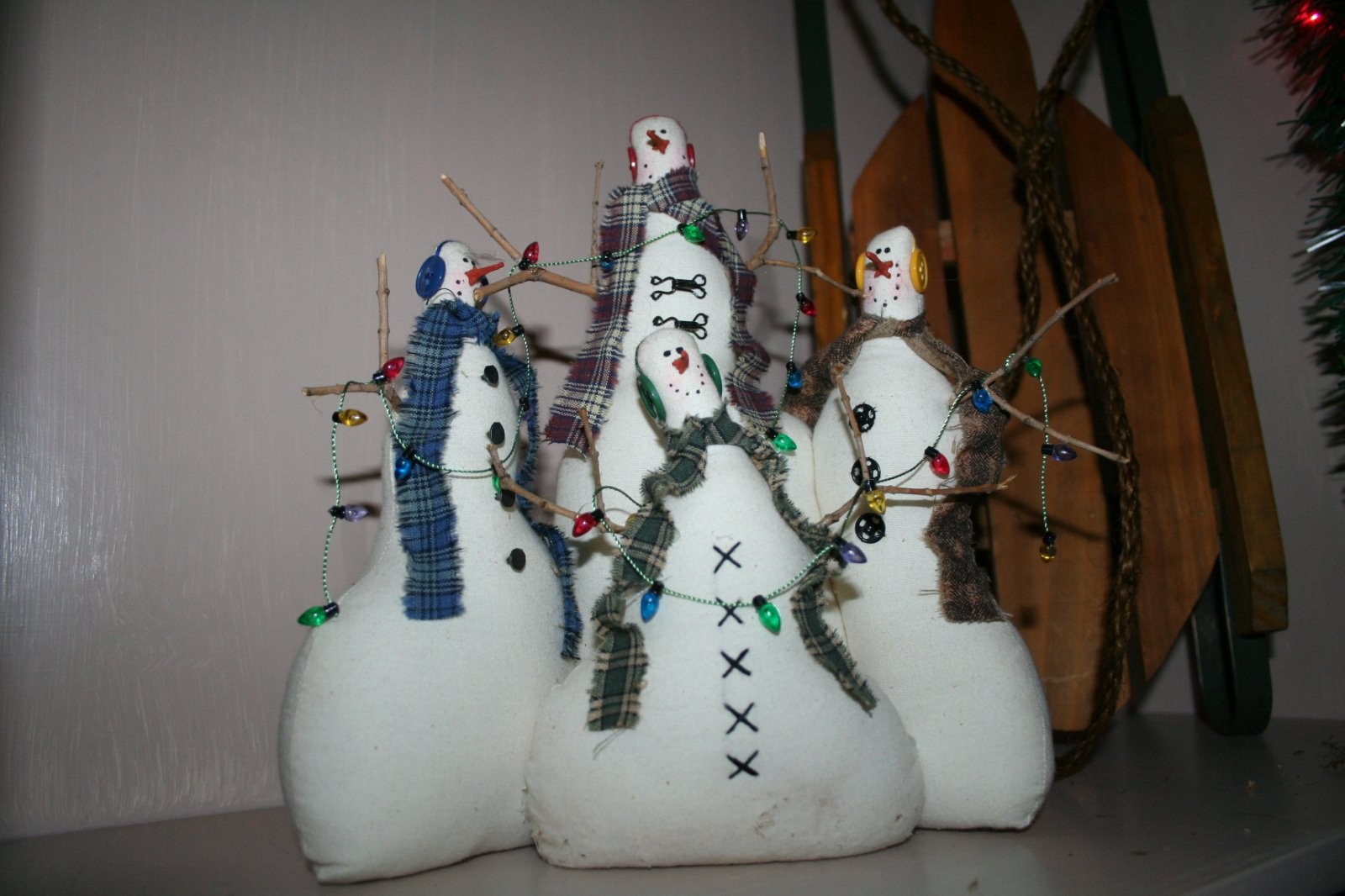This color photograph, taken indoors, vividly captures a festive Christmas decoration featuring four snowmen meticulously crafted from white sacks resembling pillows. Each snowman sports its own unique attire—a mix of colored plaid scarves and ear muffs. The snowman on the left is adorned with blue earmuffs and scarf and features four buttons on its front. Moving to the upper middle, this snowman is distinguished by double brass buttons, a red and white plaid scarf, and red earmuffs. The bottom middle snowman is dressed in green earmuffs and a matching green plaid scarf, while the one on the far right boasts orange earmuffs and an orange and black scarf. Of particular note, the upper middle snowman has X-stitches adorning its chest, and the snowman on the far right is decorated with wheel-shaped buttons. Sticks serve as arms for each of these charming figures, and they're all ringed with strands of festive Christmas lights that illuminate the scene. In the background, a sleigh can be spotted on the right, made of brown wood with several ropes, and the faint glow of a Christmas tree's red light peeks from the far corner, adding to the overall holiday cheer. The backdrop of the image is white, and the floor beneath the festive display is silver, enhancing the overall wintry atmosphere.